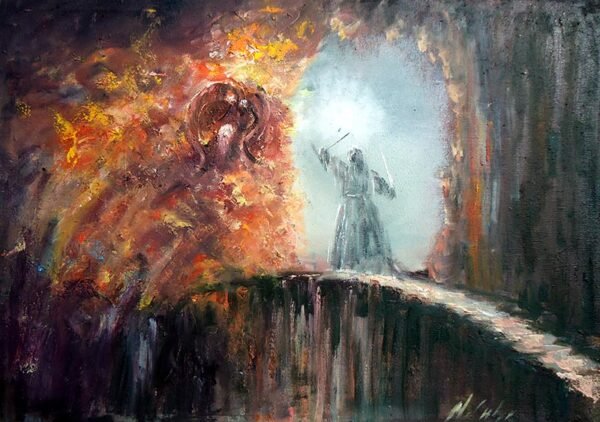The image is a stylized watercolor painting featuring a dramatic scene that invokes an abstract sense of fantasy, reminiscent of something from Lord of the Rings. At the center of the composition stands a figure, likely a wizard or warrior, with arms raised, holding a sword in one hand and gesturing with the other. The figure appears all white and is silhouetted against a gray oval background with a very light area just above them, suggesting illumination or energy. The figure is positioned on a long, abstract-looking stone stairway or walkway, which might be curved and looks cement-like. The background on the right side consists of muted shades of gray with vertical strokes, while the left side is vibrant with many shades of rust, orange, and purple, representing a monstrous entity depicted as a swirl of fiery colors. This monstrous figure has noticeable eyes and a large white mouth, with horns suggested by the shapes. The scene is framed by an overarching dark cave, blending into the sky behind the central figure. The overall palette alternates between whitish-blue hues and intense reddish-yellow tones, heightening the sense of conflict and otherworldliness.